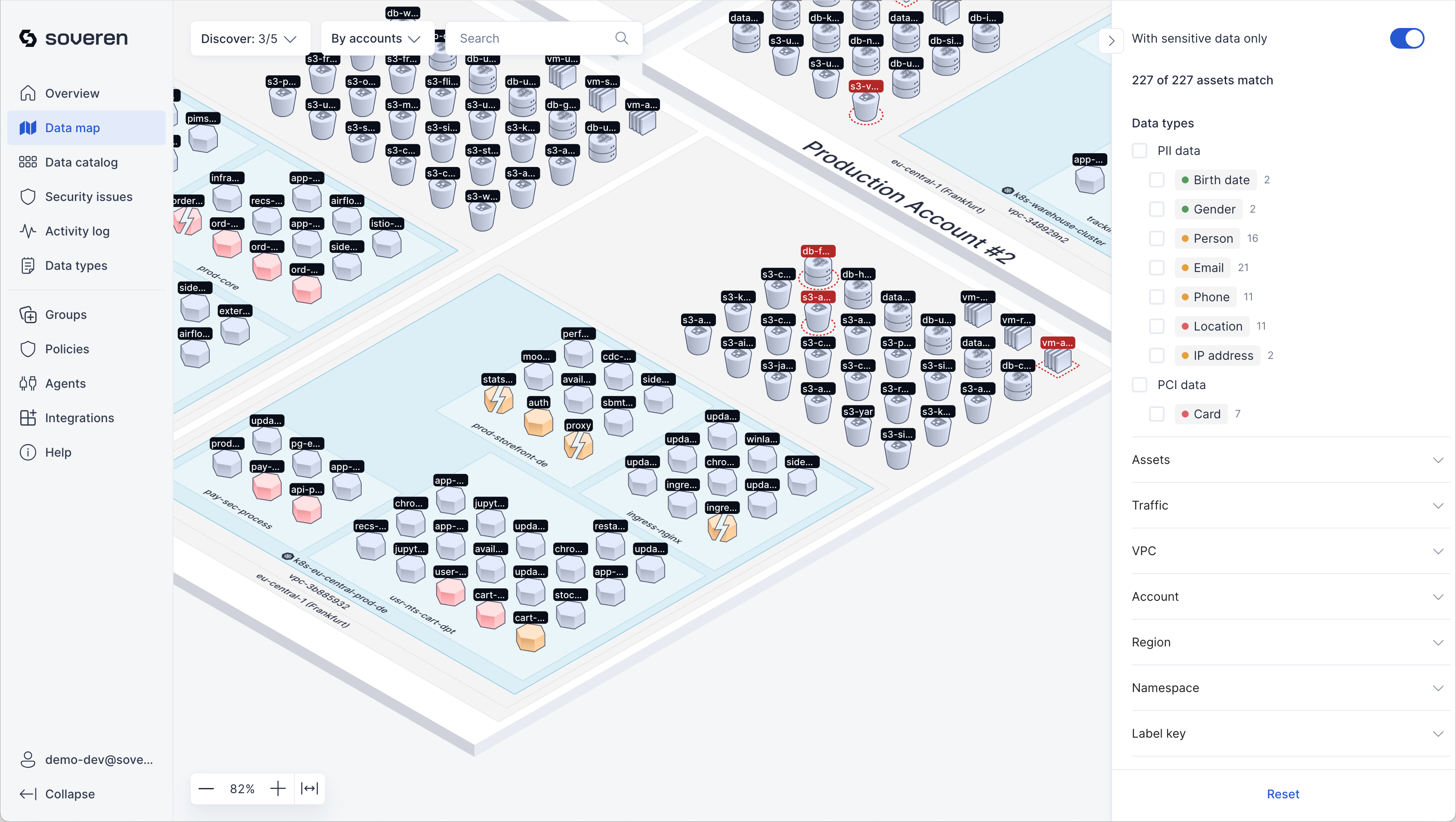Screenshot of the Sovereign Data Management Program Interface

The screenshot displays the interface of the Sovereign program, featuring a variety of navigational elements and detailed data maps. In the upper left-hand corner, the Sovereign logo is prominently displayed, consisting of a diagonally positioned "S" facing the top left corner. Down the left-hand side of the interface, a vertical menu provides options for various sections including Overview, Data Map, Data Catalog, Security Issues, Activity Log, Data Types, Groups, Policies, Agents, Integrations, and Help.

The central portion of the interface showcases a complex diagram, featuring several square boxes arranged in a diagonal pattern toward the bottom right of a larger encompassing box. These square shapes are connected and have small round or canister-like icons positioned on top of them, signifying specific data points or nodes.

In the top right corner, a label reading "Production Account Number 2" is displayed, indicating the current active account. 

On the right side of the interface, a vertical section provides detailed information about the data, highlighted with the heading "With Sensitive Data Only." It indicates that "227 of 227 Assets Match," followed by classifications of Data Types, including PII Data, Birth Date, Gender, Person, Email, Phone Location, IP Address, PCI Data, and Card. Further down, additional asset categorizations such as Traffic, VPC, Account, Region, Namespace, and Label Key are listed.